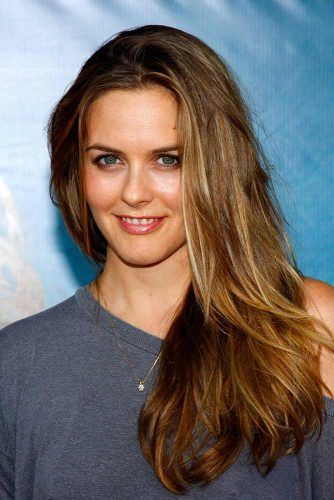This image features a close-up portrait of actress Alicia Silverstone, likely taken in her 20s or 30s. She is staring directly at the camera with a slight, confident half-smile, revealing her teeth and exuding a quiet sense of confidence. Her long, chest-length hair has a mix of brown and blonde highlights, with some of it flowing over her left shoulder and the rest cascading behind her. Alicia's light-tan skin contrasts with the delicate blue of her eyes and the pink hue of her lipstick. She wears a grayish-blue, sweatshirt-material top that obscures her right shoulder while leaving her left shoulder completely bare. Draped around her neck is a fine gold necklace with a single, dangling diamond-like gemstone. The background is a soft, blurred mix of bluish-white tones that ensures Alicia remains the central focus of this captivating photograph.